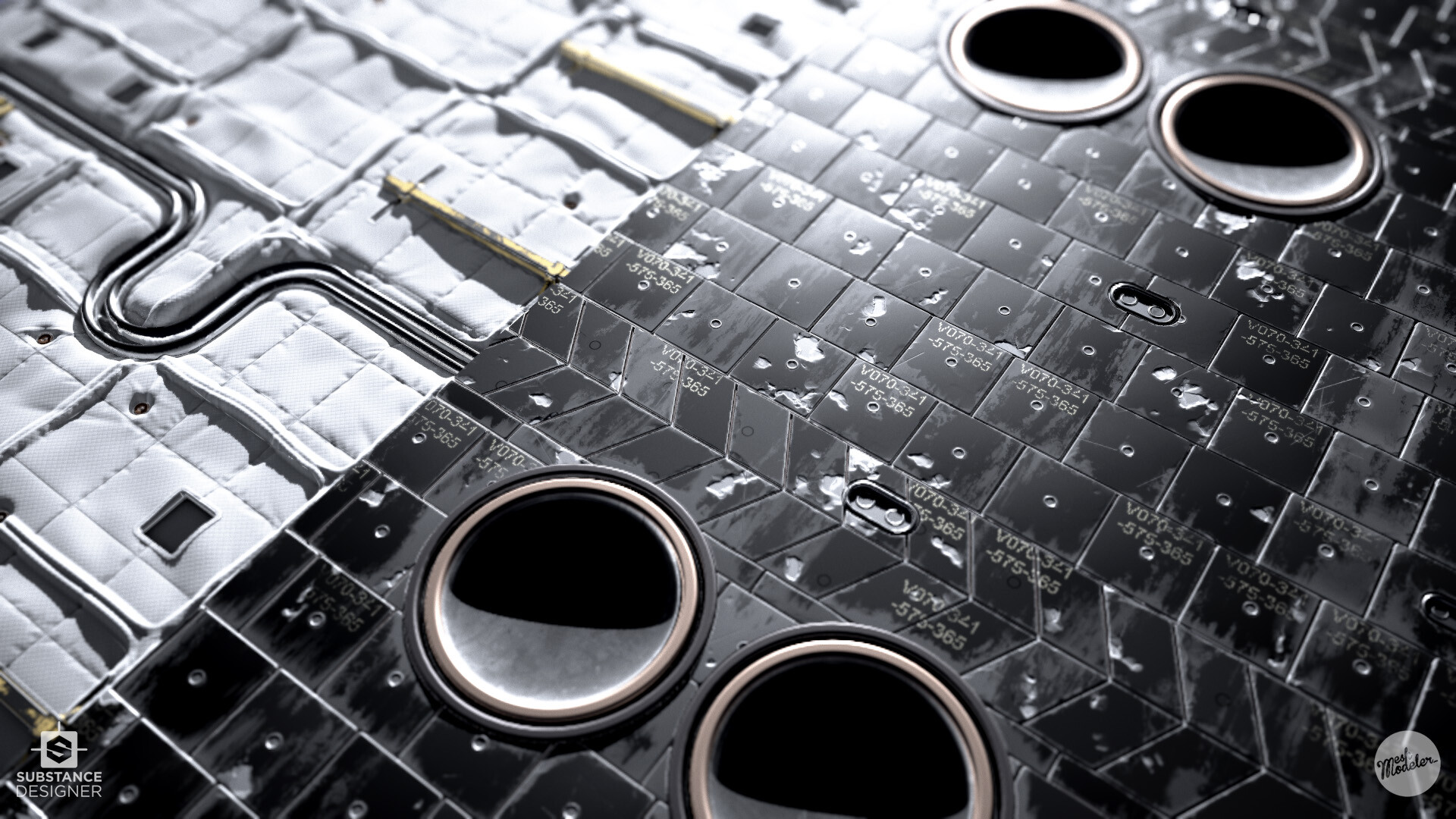The image depicts a black and white photograph featuring a detailed technological or mechanical composition, oriented in a landscape format. The scene is divided diagonally from the bottom left to the top center. On the left side of the division, a white padded surface showcases a quilted texture with visible tile-like stitching. Embedded within this area are metal components, including a stainless steel rod that curves in a U shape and gold or copper-toned pipes, along with some white wiring, creating an intricate pattern.

On the right side, the image highlights a dense array of small black tiles, possibly reminiscent of microchip surfaces or a motherboard. These tiles are meticulously arranged in a masonry brick style and bear tiny white alphanumeric codes, such as "V07054T" and "575365." A noticeable feature includes four black rings with concave centers, resembling the internal structure of subwoofers or speakers, further enhancing the intricate tech aesthetic. Some of the black tiles display minor chips, revealing a white subsurface, adding a weathered texture to the high-tech design. The photograph blends elements of realistic tech design and artistic representation.